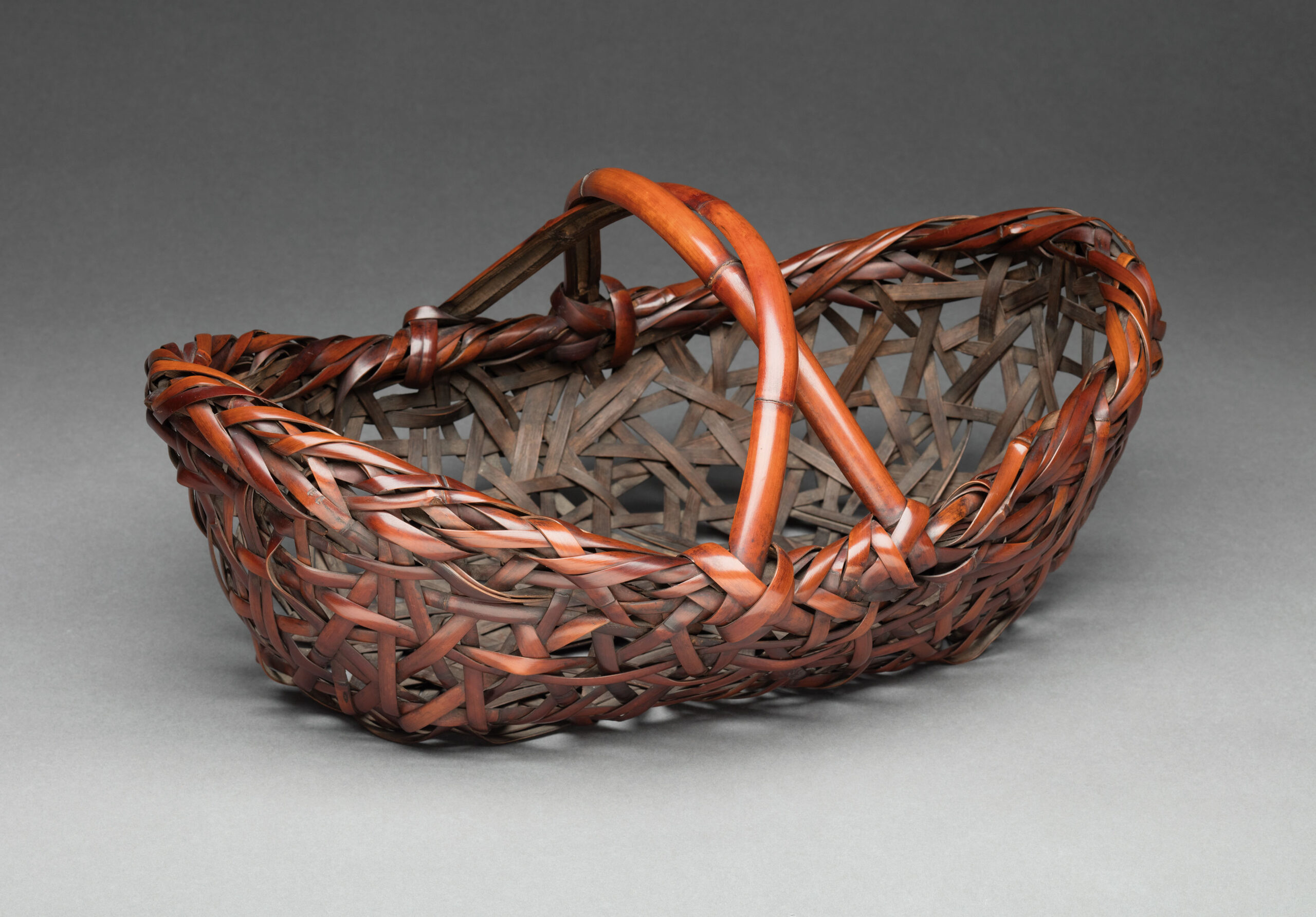This black-and-white photograph showcases a beautifully woven basket set against a gradient background that transitions from dark gray at the top to lighter shades of gray toward the bottom, culminating in white near the base. The basket itself is crafted with a high level of detail and intricacy, featuring a tight weave that speaks to its high quality. It exhibits a light brown color with subtle pink undertones, adding a unique aesthetic charm. The basket is oblong, resembling a boat in shape, and is accented with polished handles that loop over the top, giving it a slightly shiny appearance. Made possibly from bamboo, the carefully fastened ends ensure durability and functionality, making it ideal for uses such as a bread basket for hosting. The photograph captures the elegance and craftsmanship of this medium-sized basket, approximately the size of a shoe, emphasizing its beauty against the clean, minimalist background.